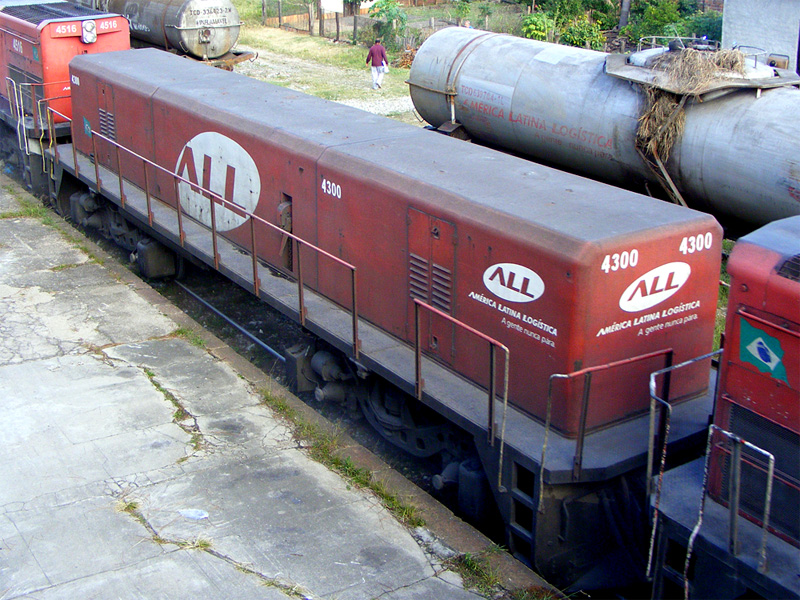The image is a color photograph, taken diagonally from the second floor of a building, capturing a scene from a train yard in Latin America. In the foreground, a faded and weathered dark red cargo train with rectangular cars stretches across the frame. The train prominently features the white oval logo with "ALL" (America Latina Logistica), along with the slogan "A GENTE NUNCA PARA" and a Brazilian flag on the side. The photograph reveals a full view of one car, as well as partial views of the adjoining cars, indicating the presence of multiple connected units. Further in the background, another train with cylindrical, silver tanker cars can be seen on a parallel track, also marked with red lettering that reads "America Latina Logistica." The overall scene exudes a sense of age and functionality, with the trains appearing old and heavily utilized.